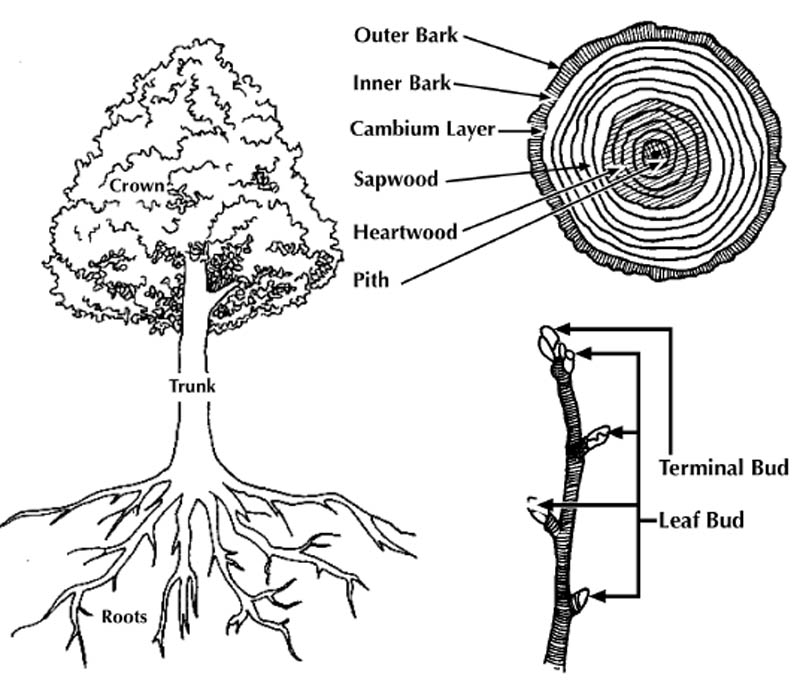This image displays a set of detailed black and white drawings focused on different parts of a tree. On the left side, there is a comprehensive drawing of a whole tree, showcasing its various parts labeled in black text. The roots are explicitly labeled at the bottom, the trunk is labeled in the middle, and the crown is labeled among the leaves. On the right side, the top section features a round cross-section of a tree trunk with multiple concentric circles, all meticulously labeled to indicate the outer and inner bark, cambium layer, sapwood, heartwood, and pith—the innermost core. Below this, there is a drawing of a branch, which is slightly curved to the left, with labels pointing to the terminal bud at the top and several leaf buds along the sides. The entire illustration is executed in clean black lines against a white background, emphasizing the anatomical details clearly.